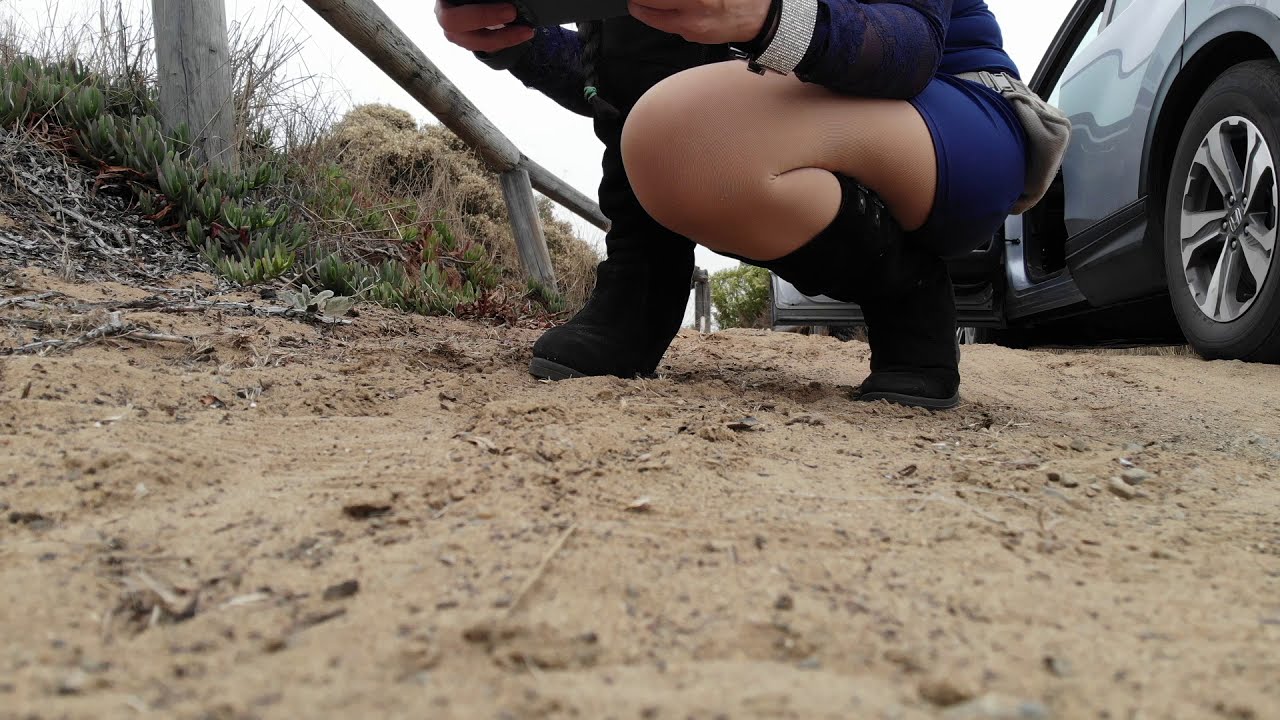In the foreground, a woman is crouched down on light brown soil interspersed with small rocks. She is wearing blue shorts and a matching blue jacket with white accents at the wrists, along with black boots. A white fanny pack is strapped around her left hip. She is kneeling with her left leg forward and appears to be holding something, perhaps a phone. Her entire posture indicates she is focused on something ahead.

To her left, the landscape shows patches of faded green grass, some light gray twigs or vines, and a wooden fence with visible vertical poles and a horizontal rail, painted in a weathered white. Adjacent to her, further right, is the lower part of a parked car, distinguishable by its silver metallic paint and clean wheels. The car door on the driver's side is open. The setting appears to be outdoors on an overcast day, with a hint of green foliage and a distant tree in the background. The overall scene looks like it was captured at a base or a similarly open area.